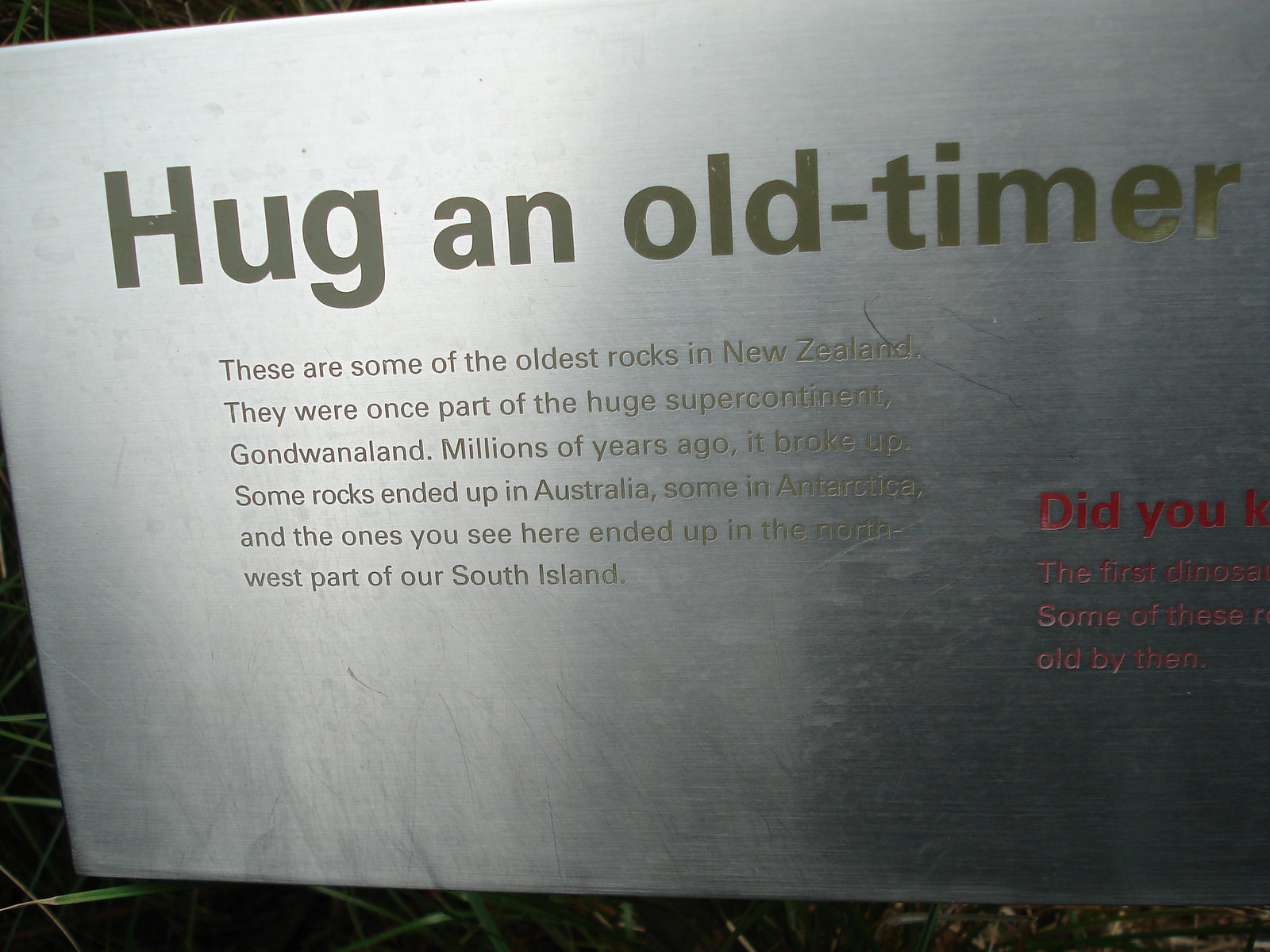This detailed image depicts a close-up of a scratched stainless steel plaque with etched text. The plaque prominently features a large title in gray font that reads "Hug an Old-Timer." Beneath this heading, smaller gray text explains, "These are some of the oldest rocks in New Zealand. They were once part of the huge supercontinent Gondwana. Millions of years ago, it broke up, with some rocks ending up in Australia, some in Antarctica, and the ones you see here arriving in the northwest part of South Island." To the right, there is partially visible red text beginning with "Did you know," followed by fragmented information about the first dinosaurs and the age of these rocks. The plaque appears to be either leaning against something or possibly affixed to a wall.